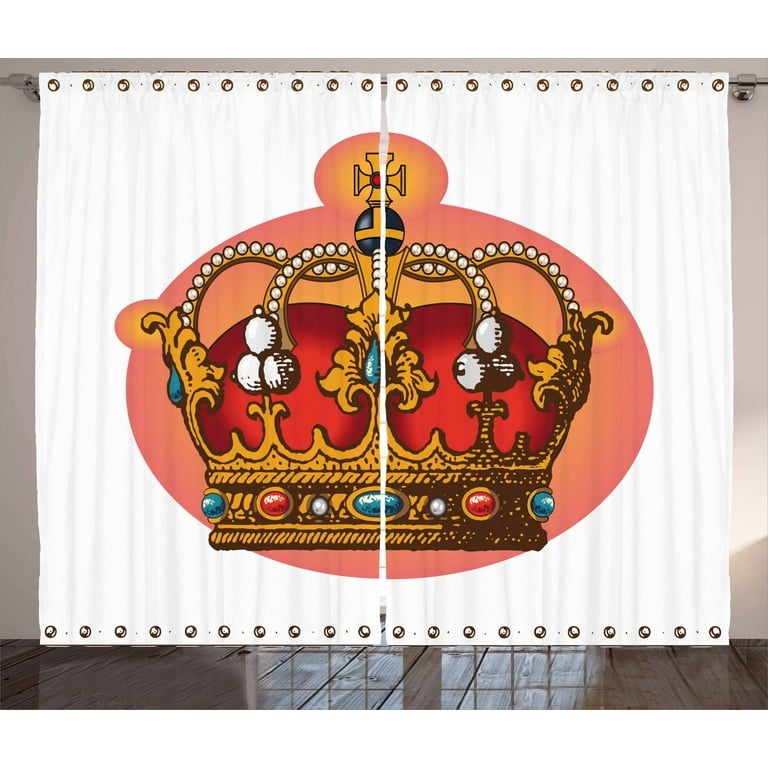The photograph depicts two separate curtain panels forming a larger cohesive image. Both panels are made of white fabric, adorned with printed graphics, and feature multiple silver metal rings along the top and bottom sides. Suspended from a silver curtain rod, the rings are not actually attached, indicating the image has been edited. The composition displays a large orange oval in the center of the curtains, housing a detailed vector illustration of a royal crown. Split by the curtain divide, the crown appears whole when the curtains are closed and halves when opened. The crown, predominantly gold, boasts a base encrusted with blue and red jewels and adorned with a scalloped gold section with arched rises studded with pearls and gemstones. The crown's apex features a gold cross, set with a ruby. The backdrop reveals a brown wooden floor reflecting a window and framed by a white wall, adding to the layered, composite nature of the image.